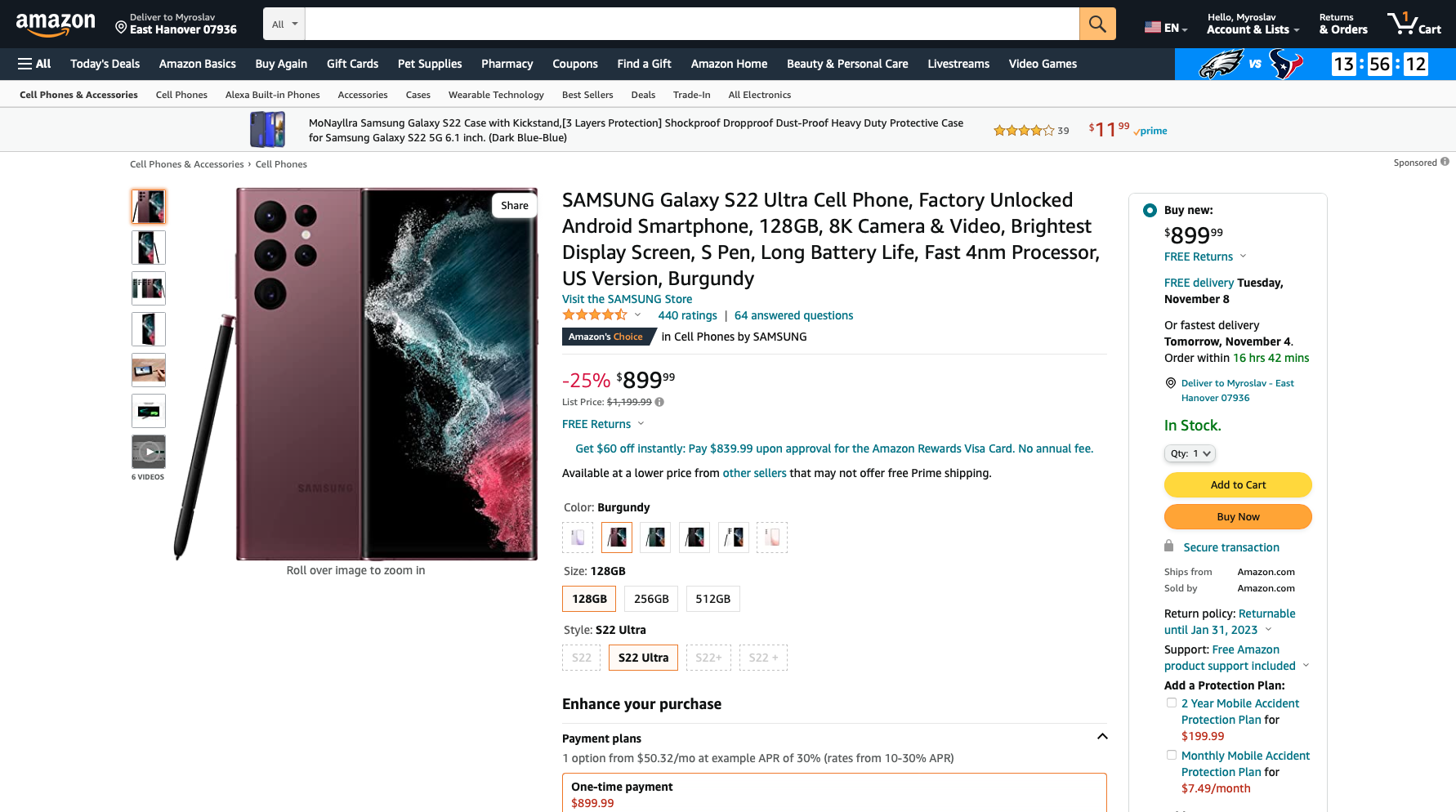This detailed screenshot of an Amazon product page features the Amazon logo, complete with its distinctive smiley arrow, situated in the top left corner. Just below the logo, there's a location indicator displaying the zip code 07936, denoted by a small GPS icon. The page's central search bar, highlighted with a magnifying glass, is flanked by an American flag icon, signifying that the language is set to English (EN). 

Underneath this header, there's a promotional banner showcasing a match between the Eagles and the Texans, with the current time recorded in military format as 13:56:12. Dominating the center of the screen is a prominent advertisement for the Samsung Galaxy S22 Ultra smartphone. Detailed information about the phone, including a high rating of 4.5 stars, is prominently displayed. The product is highlighted as "Amazon's Choice" and priced at $899. The highlighted options for the device include a burgundy color, 128GB storage capacity, and the S22 Ultra model. The right side of the screen features essential purchase buttons, including "Add to Cart" and "Buy Now."